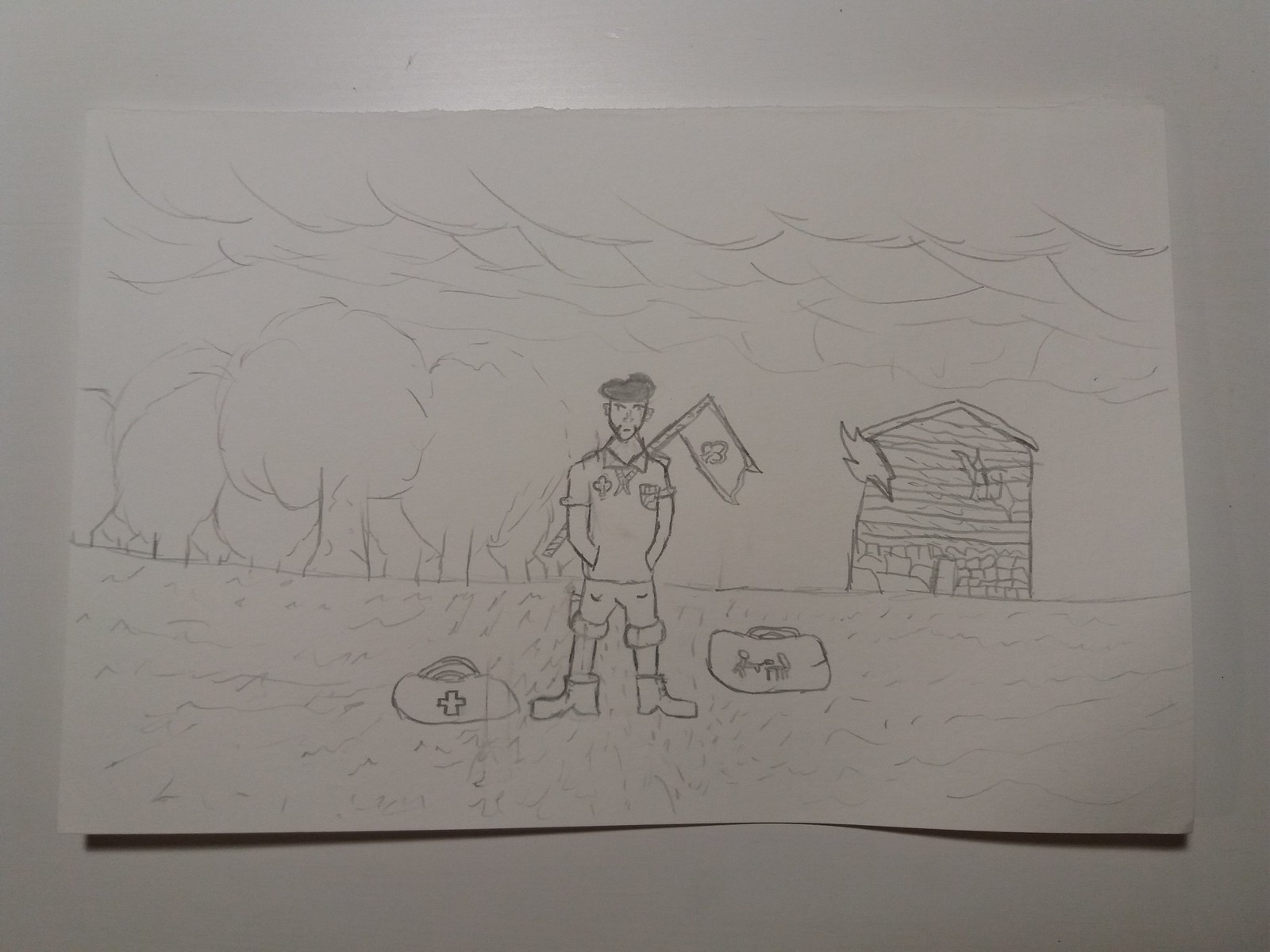This black-and-white photograph, captured in landscape format, features an A4 piece of white paper positioned horizontally on a white surface. The image on the paper is a rudimentary pencil sketch, likely created by an amateur, perhaps a child. The sketch portrays a bearded man wearing a beret, standing in a field. He has a flagpole diagonally strapped to his back, displaying a flag with a clover or fleur-de-lis symbol. The man, who also sports a kerchief around his neck, has both hands in his pockets. At his feet lie two bags; one appears to be a medical kit marked with a cross, while the other bears indiscernible doodles. To the man's right, a building, seemingly wooden, is depicted with flames emerging from it. To his left, several trees shape the horizon. Above, the sky is filled with swirling lines indicating clouds. The photograph is unevenly lit, with the primary light source coming from the top, casting a dim illumination over the scene.